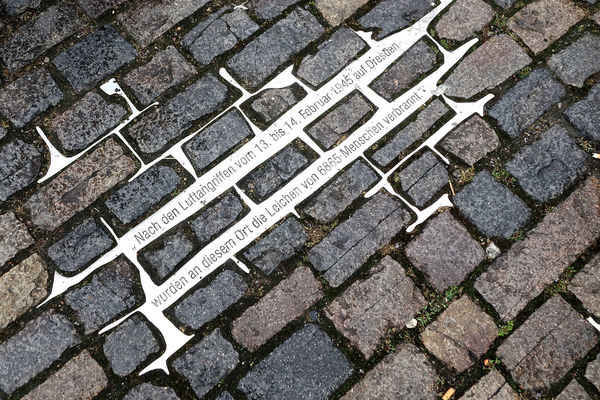This image is a close-up photograph of a cobblestone pathway, where the stones, a mixture of gray and brown, are arranged in rows with irregular gaps filled with dirt and moss. The cobblestones are rectangular or square and appear to be set at an angle. The central focus of the image is an intriguing section where the spaces between the stones are filled with a conspicuous white substance, which could be paint or plastic. This section contains text in German that reads, "Nach den Luftangriffen vom 13 bis 14 Februar 1945, Dresden," which references the air raids on Dresden from February 13 to 14, 1945. The white background and text contrast sharply with the natural appearance of the stones, suggesting that the image might be digitally edited. Near the bottom right corner, the stones are closer together with visible grass or moss growing between them, further highlighting the distinct and possibly altered nature of the central text area.